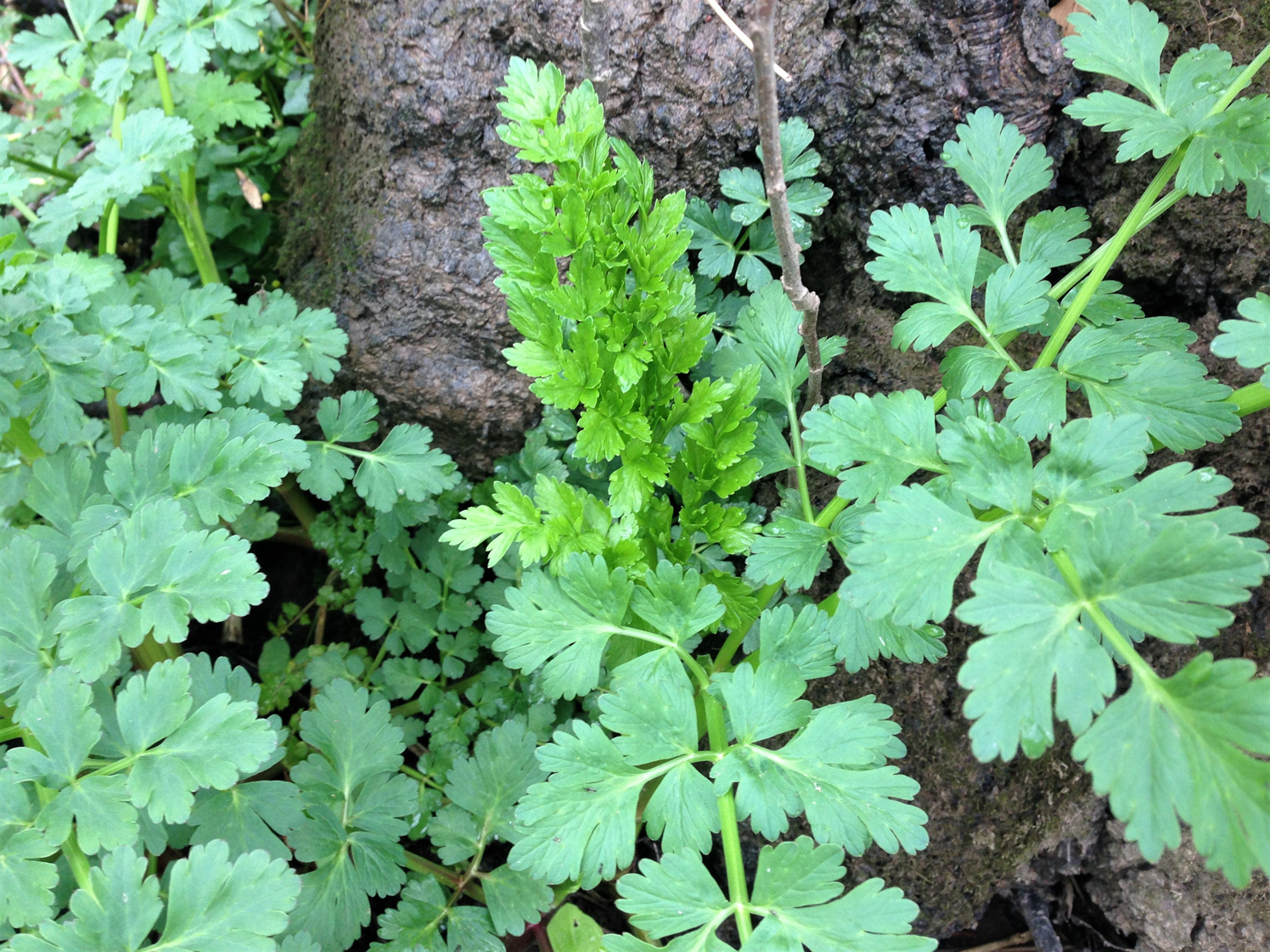The photograph depicts a close-up view of plants, most likely cilantro or parsley, growing in a natural area. The greenery features distinctive leaves that resemble the three-leaf pattern typical of parsley or cilantro, each set emerging from green stems. The scene captures the plants thriving amid a dark brown, earthy ground, which might be composed of dirt or tree bark at the base. The lush green leaves contrast sharply with the surrounding brown ground, and the image appears to be taken from above, possibly showing the plants populating the left, center, and extending to the right over a rocky surface or cliffside.